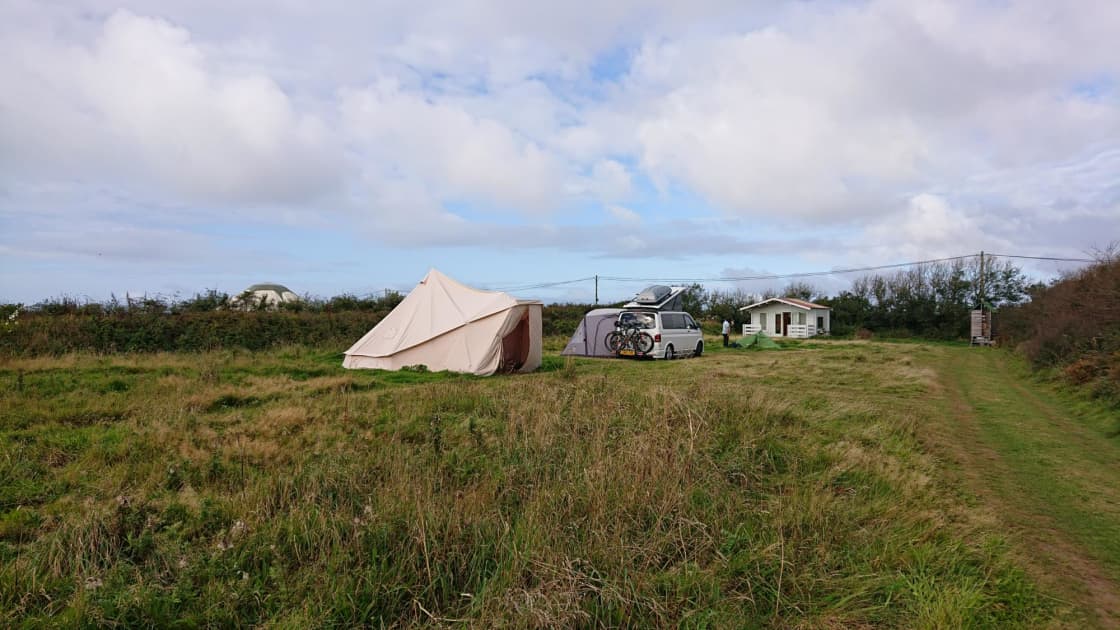This image is a detailed color photograph taken outside on a cloudy day in a large field with patches of green and brown grass. Dominating the scene is a small white house with a red roof, featuring a cozy porch with white railings. To the right of the house, a man is standing in the distance.

In front of the house, there is a white van with a luggage pod on top and two bicycles attached to the back. The van's rooftop is popped open, likely revealing a solar panel setup or an elevated tent. To the left of the van, an extension tent is set up, leading to a large white tent with one side open, facing the field. This open tent is flanked by a collapsed green tent off to the side.

A power line stretches across the field behind the house, and a dirt path can be seen to the right, cutting through the tall brush and green grass. In the horizon, the sky appears mostly overcast with thick gray clouds, interspersed with occasional patches of blue sky, giving the scene a subtly melancholic yet picturesque atmosphere.